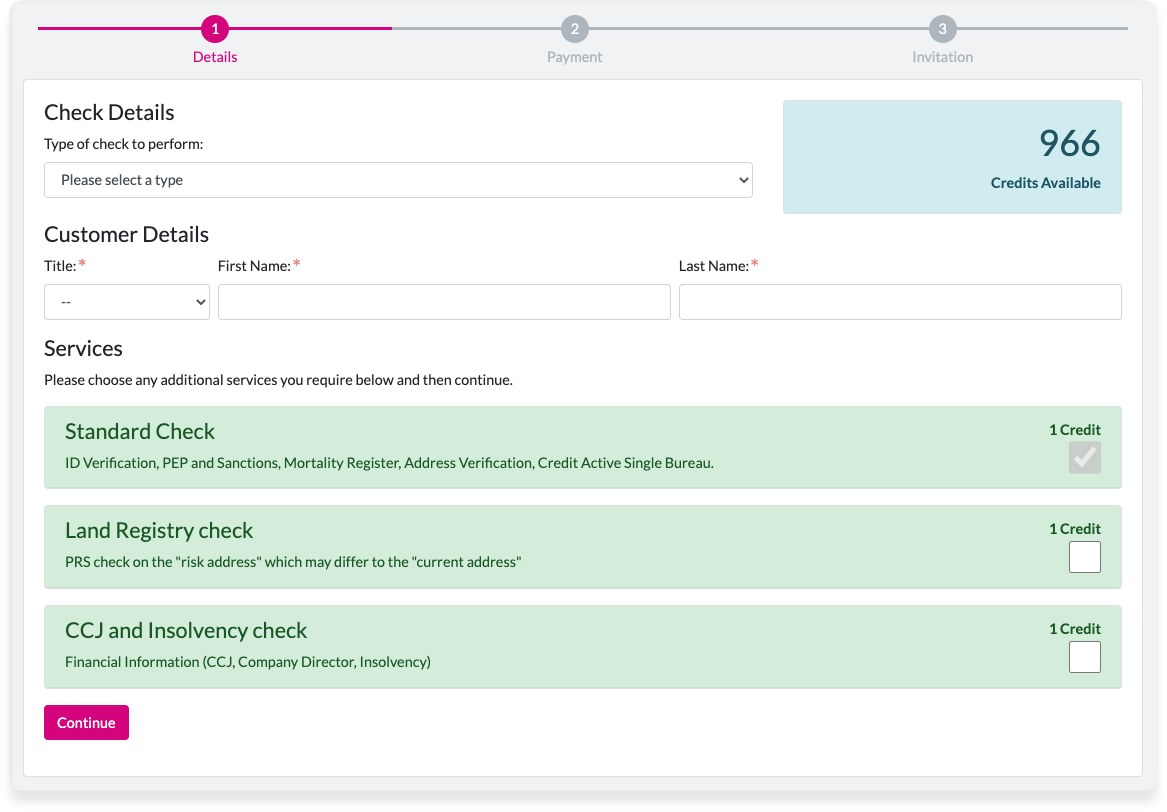A screenshot features a clean white background with an interface populated by various elements. At the top, a series of four circles are numbered "1, 2, 3, 1," with the first circle highlighted in pink and the remaining circles in gray. The heading "Check Details" appears, followed by the subheading "Type of Check to Perform." Below is a selection box with 966 credits available displayed prominently to the right. This area is bordered by a dark blue and light blue rectangle.

The middle section, titled "Customer Details," includes fields labeled "Title," "First Name," and "Last Name," each marked with a red asterisk to indicate mandatory information.

Further down, the "Services" section invites users to "Please choose any additional services you require below, and then continue." Here, three options are presented:

1. "Standard Check" with a brief description, accompanied by a checkbox that is ticked, indicating it requires one credit.
2. "Land Registry Check" with a checkbox that is unticked, also requiring one credit.
3. "CCJ and Insolvency Check" with an unticked checkbox, necessitating one credit.

Finally, at the bottom left of the screen, there is a pink rectangle containing the word "Continue" in white text.